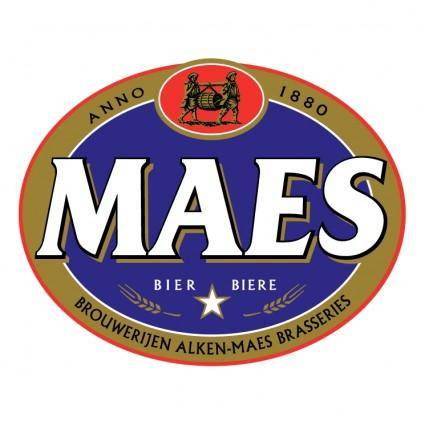The image depicts an oval-shaped beer label, predominantly outlined with a red line, followed by a gold border. At the very top of the label, it features a smaller red circle containing a gold emblem of two men carrying a beer keg on a beam secured by ropes. Above this emblem, the word "Anno," followed by "1880," is prominently displayed, suggesting the founding year of the brand.

The central part of the oval label is a dark blue background with the large white text "MAES" boldly stamped across its center. Directly below this text, in smaller white font, are the words "B-I-E-R" on the left and "B-I-E-R-E" on the right, meaning "beer," with a white star outlined in gold positioned between them. Additionally, on either side of the star are gold hops.

Encircling the bottom part of the gold border is some text in a foreign language, possibly German, which adds to the label's intricate design. This detailed and historical label is indicative of a classical beer brand.